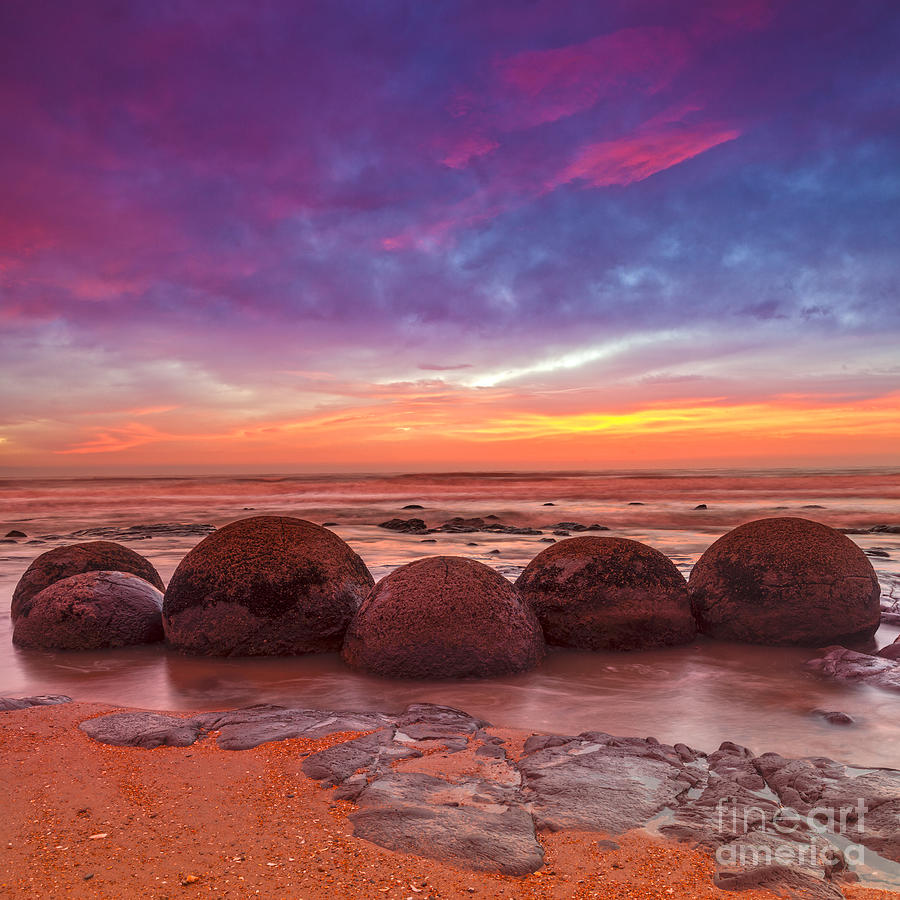An enchanting image captures the serene beauty of an ocean shore at sunset, showcasing a rocky shoreline with the beach's sand appearing vividly orange. Dominating the scene are six remarkably spherical boulders, perfectly round and arrayed just a few feet into the water, creating an almost surreal and unnatural visual. These boulders display an array of colors from dark browns and grays to highlights of orange, reflecting the vibrant hues of the setting sun. The expansive ocean extends to the horizon, blanketed in waves. Above, the sky transitions from a bright orange and yellow near the horizon to light blue, dark blue, and pink, forming a stunning gradient that adds depth and beauty to the scene. The 'Fine Art America' watermark in the bottom right corner suggests this image's professional and artistic caliber.